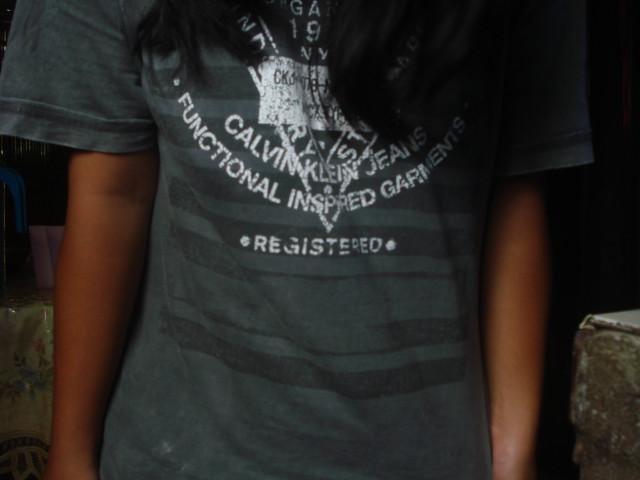In this image, we primarily see the torso of an African-American female, identifiable by her arms and the long black hair partially covering her chest. The main subject of the image is a dark green, short-sleeved shirt with horizontal stripes in a darker shade of green. On the front of the shirt, a white design featuring an upside-down triangle is visible, with some text overlaying it. The text includes "Calvin Klein Jeans," followed by "Functional Inspired Garments," and the word "Registered" with a dot on either side. The background appears to be very dark, possibly made of stone or concrete, making it difficult to discern specific details. Part of the setting behind her includes a dining area with a table and some cups, as well as a counter.